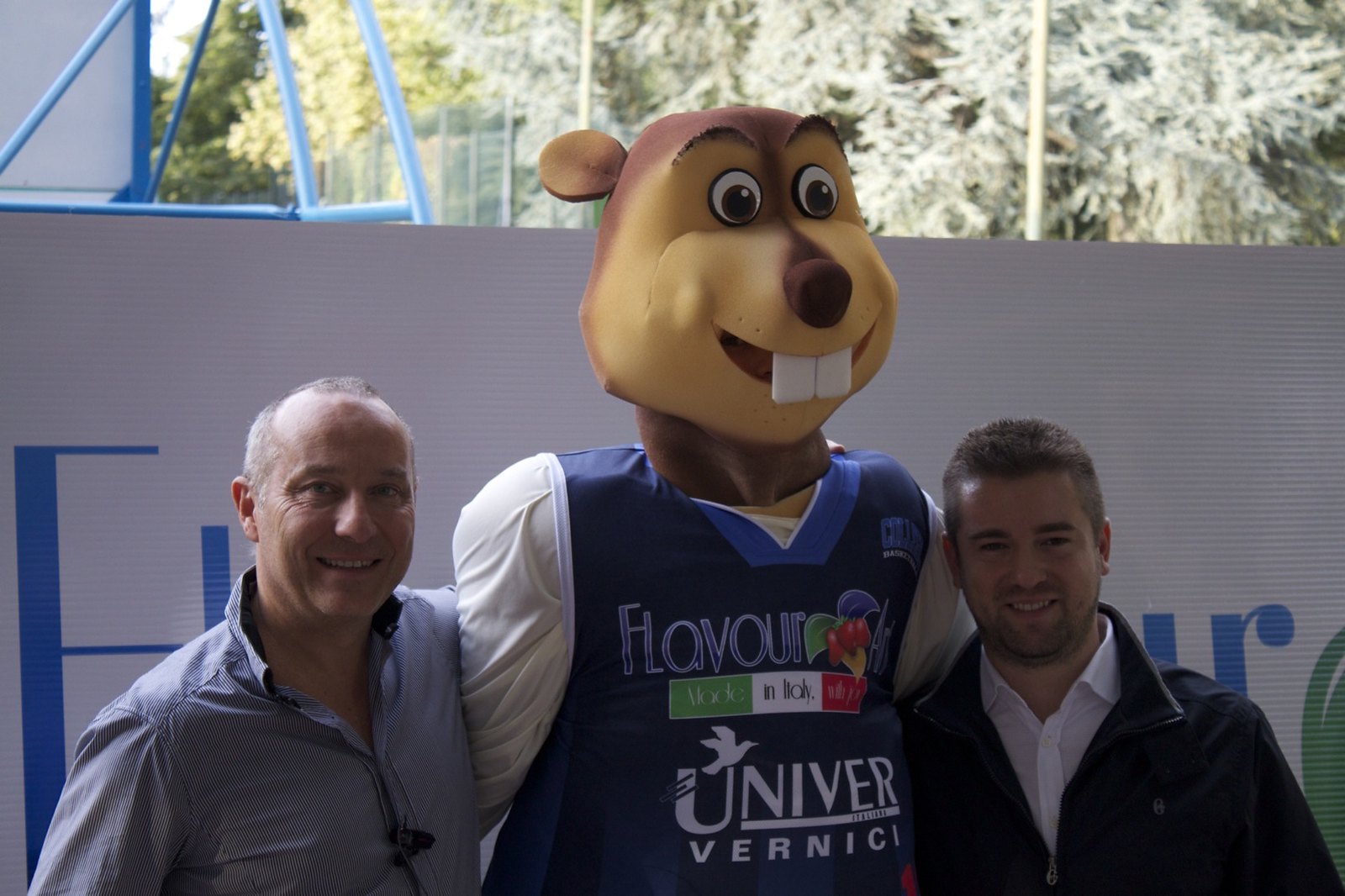The photograph depicts an outdoor scene featuring three individuals standing closely together. In the center is a person dressed as a mascot, resembling a groundhog or beaver. The mascot costume has a large, brown head with two protruding front teeth and a brown nose. The mascot is wearing a white and blue outfit with the word "Flavor" prominently displayed on the blue jersey. The jersey also features Italian flag colors (green, white, and red) and text that reads "Univer Vernici."

To the left of the mascot stands a man with short gray hair, smiling. He is wearing a blue collared shirt, potentially with a microphone attached to it, as if he were speaking or announcing. To the right of the mascot is another man with short brown hair and some facial hair, also smiling. He is dressed in a white shirt underneath a dark jacket. 

In the background, several details can be noted: there is a white display board with blue writing on it, though the text is largely obscured. Further back, trees are visible under the bright sunlight, contributing to the overall cheerful ambiance of the image.